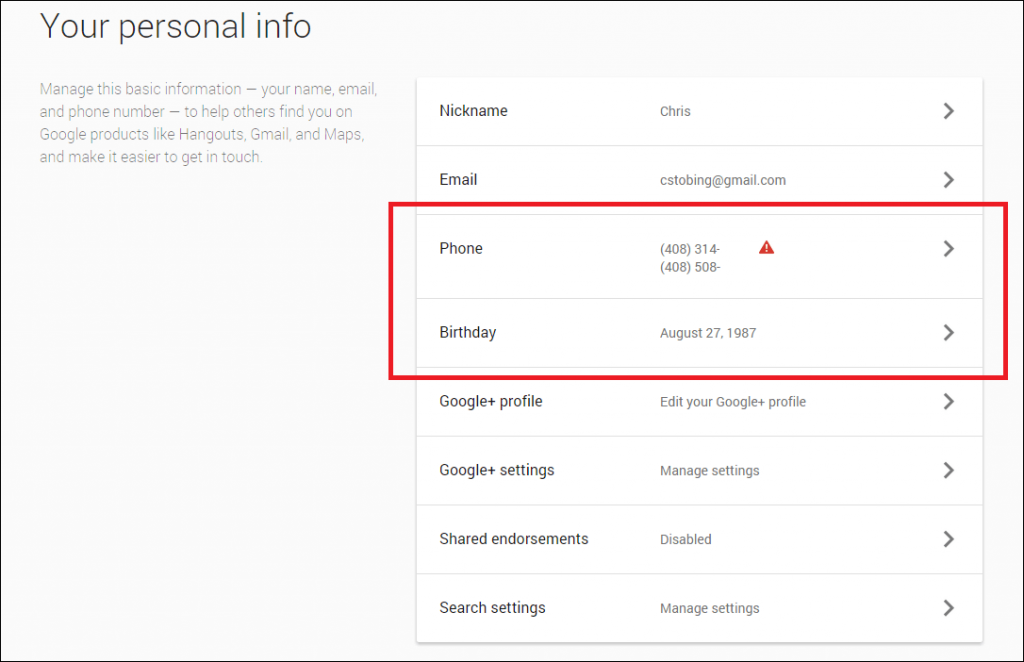This image features a light blue background with a large blue box outlined by a thin black line. At the top of the box, the text reads: "Your personal info. Manage this basic information, your name, email, and phone number to help others find you on Google products like Hangouts, Gmail, and Maps, and make it easier to get in touch."

On the right side of the blue box, there is a large white box segmented by thin blue lines into various sections:

1. The first section is labeled "Nickname," displaying the name "Chris" with a right arrow next to it.
2. The next section shows the email address "cstobing@gmail.com" also accompanied by a right arrow.
3. Below that is a highlighted area outlined in a bold red box containing "Phone" and "Birthday" details. The phone number is displayed alongside a red triangle with an exclamation point, implying an alert or error. Further down, the birthday information is listed as "August 27, 1987," with another right arrow.
4. Following these details, there is a section for "Google Plus profile," with an option to "Edit your Google Plus profile" and a right arrow.
5. The "Google Plus settings" section allows users to manage their settings, indicated by the text "Manage settings" and another right arrow.
6. The "Shared endorsements" section is marked as "Disabled," with a right arrow next to it.
7. Finally, the "Search settings" section offers the ability to "Manage settings," accompanied by a right arrow.